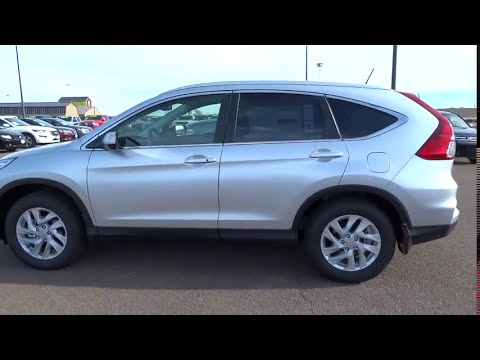The image depicts a silver SUV with black wheels, prominently positioned in the center and facing towards the left, with its hood slightly cropped out of the frame. The SUV, which seems unoccupied and not for sale, features hubcaps resembling twirling flower decorations and large brake lights near the top of the rear windshield. It appears to be parked in a paved parking lot, possibly similar to one you might find at a grocery store, surrounded by other vehicles including a black car, a white car, and a maroon car, with another black car positioned to the right of the silver SUV's rear. The background reveals several brown, barn-like buildings, some utility poles, and a bright, clear sky without visible sunlight. The image is bordered by black horizontal bars at the top and bottom.